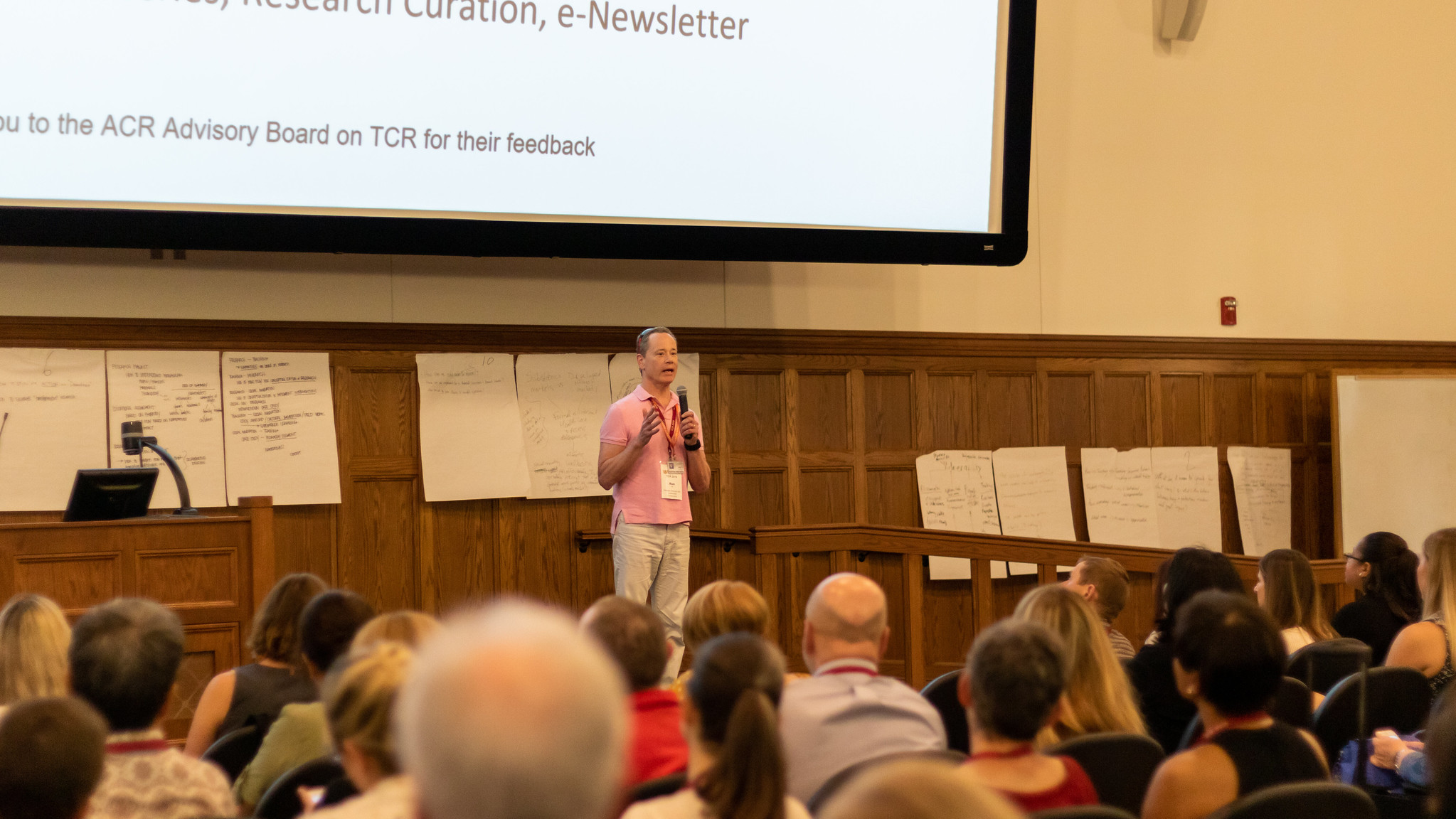The photograph features a middle-aged man, likely in his 40s, delivering a lecture at the front of an old, wooden-paneled lecture hall. The man, who appears to be a professor, is dressed in a short-sleeve pink polo shirt, khaki pants, and a lanyard around his neck. He holds a microphone in one hand, addressing an audience seated before him. The image captures the backs of the audience's heads, totaling at least three or four visible rows, suggesting a packed house. Behind the speaker, several large sheets of white notepad paper covered in illegible marker scribbles are taped to the wall. Above the speaker, a large projection screen displays text, with the only readable portion stating "e-newsletter to the ACR advisory board on TCR for their feedback." To the right of the speaker, there is a podium equipped with a laptop and another microphone. The room's upper walls are painted yellow, contrasting with the wooden paneling below.